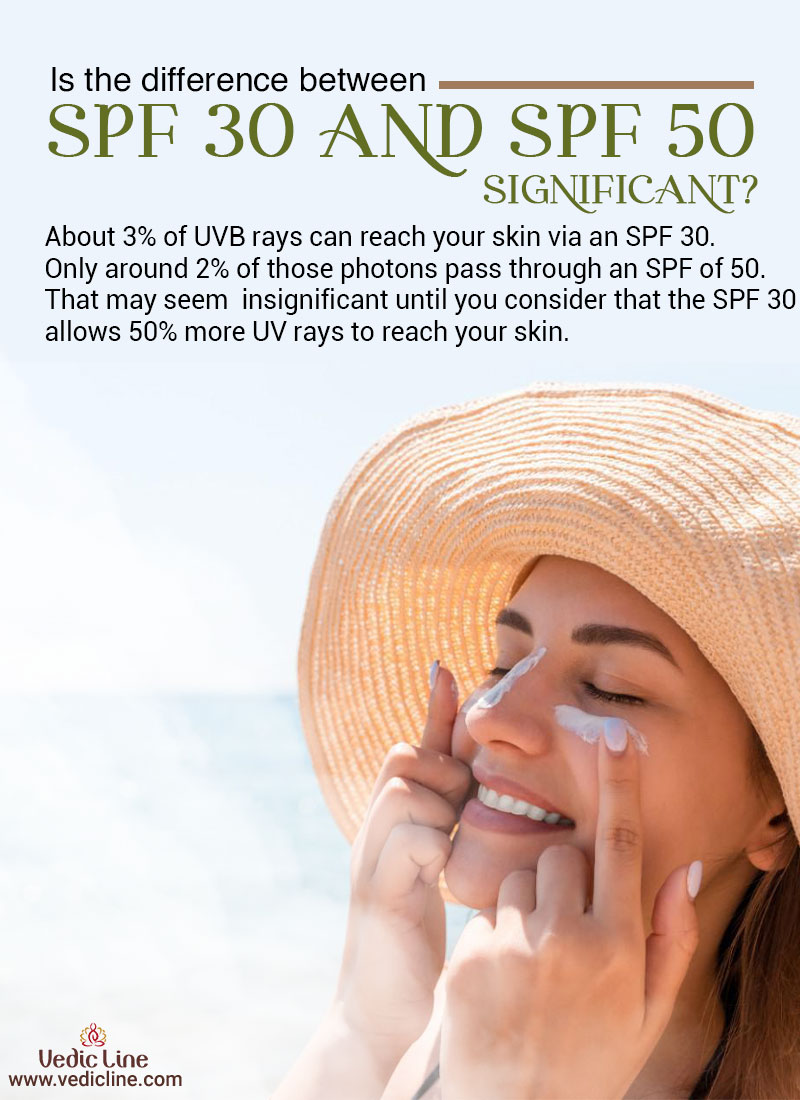The image is a full-page advertisement for skincare, featuring a Caucasian woman in the bottom right corner who is smiling and applying sunscreen. She is wearing a wide-brimmed, orange beach hat and has brown hair. The sunscreen is visibly spread on the bridge of her nose and under her eyes, with her eyes closed as if she is enjoying the moment. The top of the ad reads, "Is the difference between SPF 30 and SPF 50 significant?" in green and black text. Below, it explains, "About 3% of UVB rays can reach your skin via an SPF 30. Only about 2% of these photons pass through an SPF 50. That may seem insignificant until you consider that SPF 30 allows 50% more UV rays to reach your skin." To the bottom left of the image, there is a logo and the text "VedicLine www.vedicline.com".